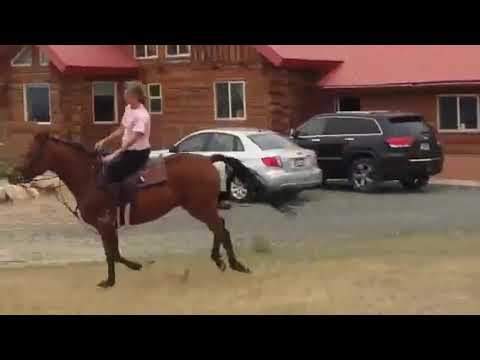This outdoor daytime photograph showcases a woman with grayish hair riding a brown horse with distinctive black socks, mane, and tail. The woman is wearing a pink short-sleeved shirt and black pants and is positioned on the left side of the image. The horse appears to be trotting across a grassy area, which transitions into a light sand dirt runway and then a paved parking lot. Behind them, a black SUV and a white or silver sedan are parked in front of a two-story, brown-wood house with red gabled rooftops and multiple windows—six are visible. The house's details include red slanted roofs and a log-cabin style. The image is framed with black bands on the top and bottom, making it longer than it is tall, and there is no visible text within the picture. The overall setting suggests a calm moment captured on a farm in the middle of the day.